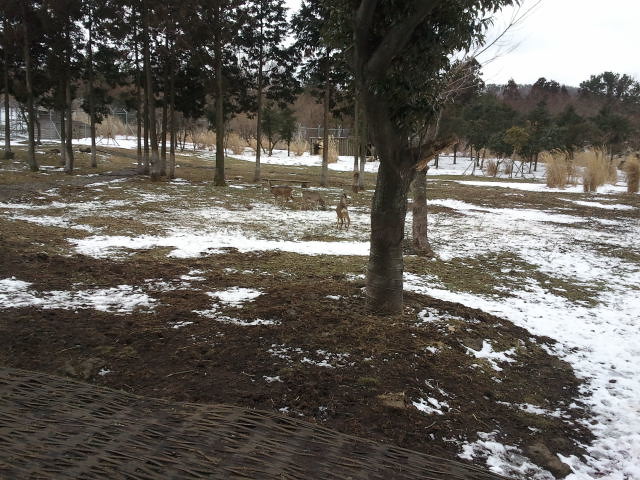The image depicts a winter scene in a park-like area with a large, predominantly brownish field interspersed with patches of melting snow. The snow appears as a light cover, allowing the underlying dirt and dried grass to show through. Towering pine trees with greenish-brown hues dominate the landscape, while more trees with sparse, dark branches stand in the middle of the field. Towards the front, a dark walkway—possibly a sidewalk or road—cuts through the scene. The distant background features yellowish bushes, more trees, and the faint outline of a wire fence. The sky is overcast with a flat, hazy layer of white clouds. In the middle of the field, small figures—likely running dogs, though too distant to distinguish clearly—add a touch of life to the tranquil winter setting.